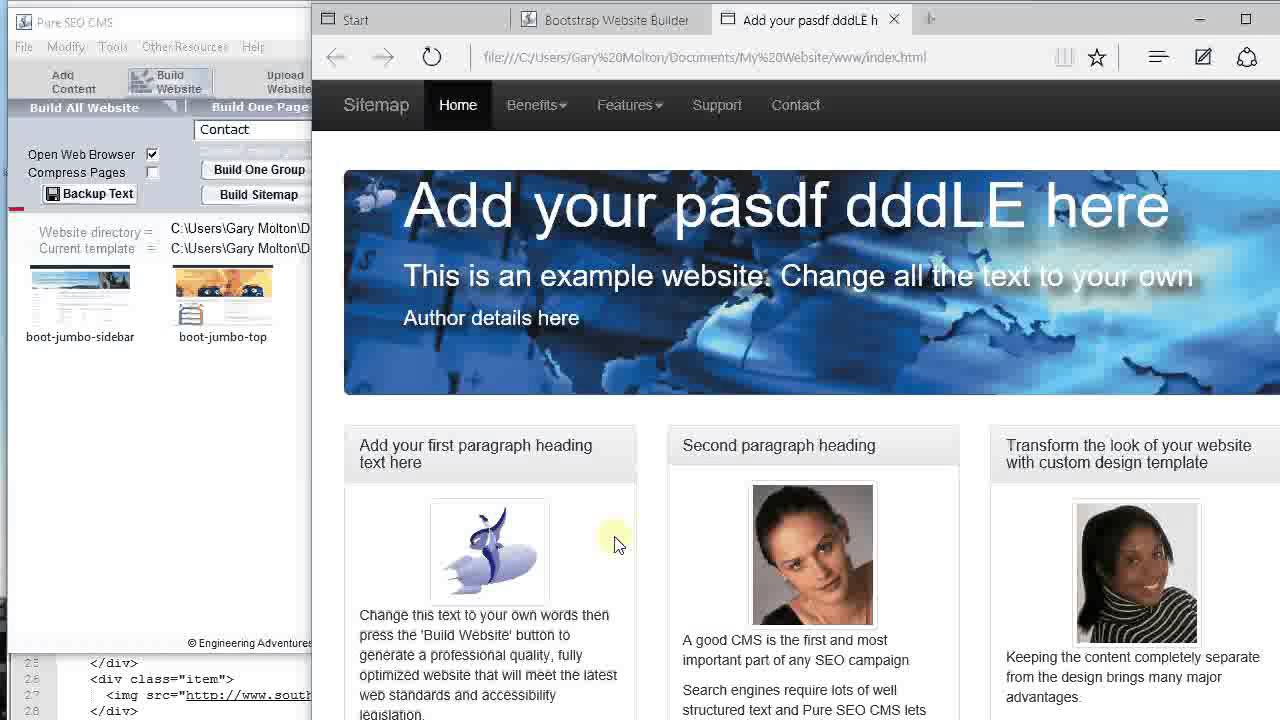Screenshot Description:

The image is a detailed screenshot of a desktop where multiple application windows are open. The primary focus is a web browser displaying a web page being built using the Bootstrap website builder. The main section of the page includes placeholder text such as "add your pass then DLL here" and "change all the text to your own author details here," written in white against a somewhat abstract blue background resembling a map.

Below this, the page is divided into three boxes. The leftmost box features the text "add your first paragraph heading here" above a small picture, with the additional instruction "change this text." The middle box has a picture of a person and a heading stating "second paragraph heading," followed by the text "a good CMS is the first step and most important part." The rightmost box reads "transform the look of your website with a custom design template" and includes another picture of a person, along with the advice to "keep the content completely separate."

In the secondary window beside the web browser, there appears to be a file explorer or text editor displaying various tasks related to web development. These tasks include "open web browser," "compress pages," "backup text," and a glimpse of some HTML code. Additionally, a portion of a spreadsheet is visible at the bottom of the screenshot, indicating that multiple tools and files are being utilized in the web development process.